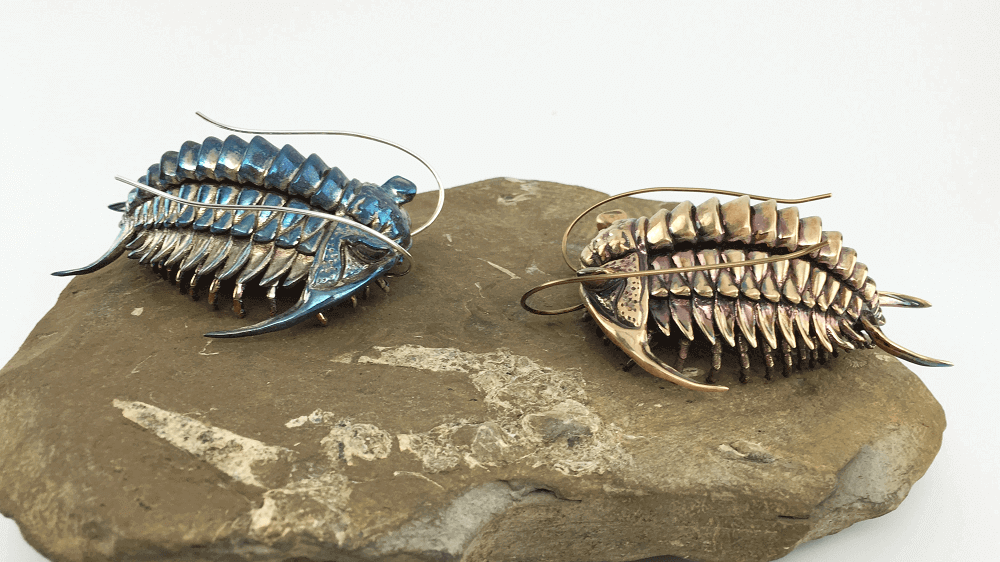The horizontally aligned rectangular image depicts two intricate metal sculptures, resembling fossils of beetle-like insects or crustaceans, displayed on a contrasting rock surface. The background is a very light gray, almost white, with no border. Positioned on a dark brown rock with light brown spots, the two sculptures face each other. The sculpture on the left is primarily blue with vertical rows of blue crystals, emulating a skeletal, segmented body with three distinct rows of short crystals. It has tall, curved antennae that extend towards the back past halfway down its body and two small tail-like appendages at the back. The right sculpture, predominantly in shades of gold and brown, mirrors the intricate detailing of its counterpart with its own segmented, spiked exoskeleton, long curved antennae, and bifurcated tail. The meticulous craftsmanship highlights the sharp, pointed features and the horn-like structures on each side of their heads, creating a visually arresting representation of these metallic fossilized creatures.